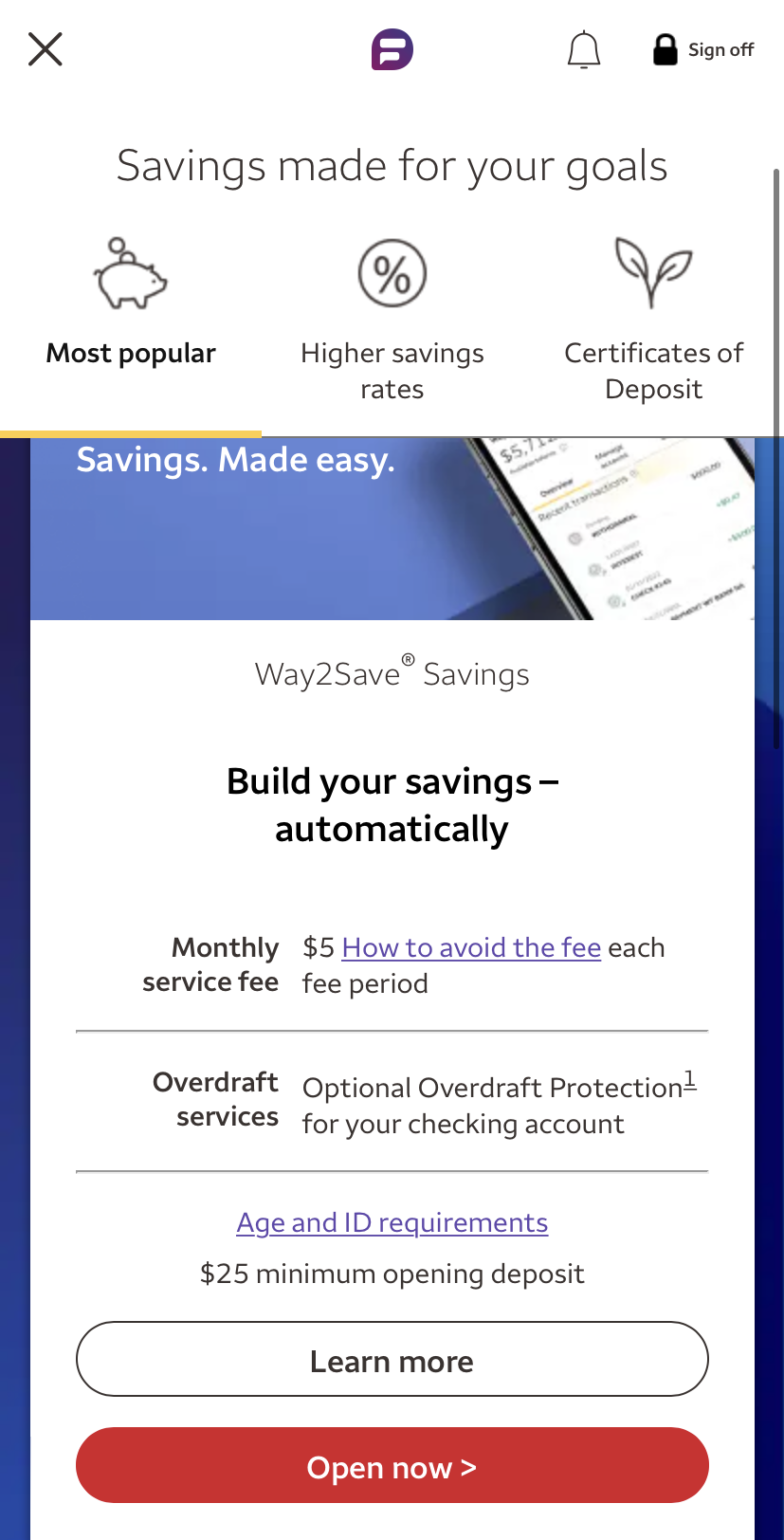This image is a cropped screenshot from a mobile banking app. Displayed prominently at the top center, in large grey letters, is the phrase "Savings made for your goals." Directly below, three icons are horizontally aligned conveying different saving options: 

- To the left, a piggy bank icon labeled "Most Popular."
- In the center, a percent icon with the phrase "Higher Savings Rates" below it.
- To the right, a little leaf icon labeled "Certificates of Deposit."

Following these icons, there's a large rectangular box showing partially scrolled content. At its top, partially cropped out, it reads "Savings made easy." The visible content includes:

- A heading "Ways to Save Savings" encouraging users to "Build your savings automatically."
- The monthly service fee, overdraft services, and corresponding descriptions. 
- A clickable blue hyperlink labeled "Age and ID requirements," centered within the box.
- A centered note "25 minimum opening deposit."
- Below the text, two horizontally centered buttons:
   - The top button, "Learn More," is styled with a white background and black letters.
   - The bottom button, "Open Now," features a red background with white letters and an arrow pointing left, positioned to the right of the word "Now."

Each section and detail are organized to guide the user through understanding and taking action to open a savings account.